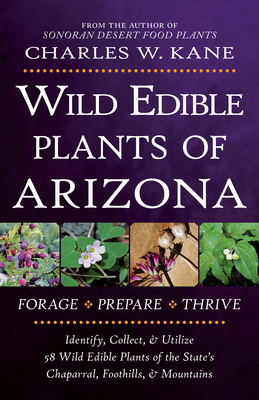The cover of the book "Wild Edible Plants of Arizona" by Charles W. Kane features a gradient background that transitions from dark purple in the top right corner to black towards the bottom left. At the top in white text, a note from the author of "Sonoran Desert Food Plants" introduces the book. Below that, Charles W. Kane's name is prominently displayed in white, flanked by approximately three dozen orange circular dots. The title "Wild Edible Plants of Arizona" appears in large white letters. Centrally placed are four square images depicting various wild edible plants—including ones with purple berries and white flowers. Below these images, a black banner bears the phrases "Forage, Prepare, Thrive, Identify, Collect, and Utilize 58 Wild Edible Plants of the State's Chaparral, Foothills, and Mountains," alongside more orange dots. Despite the cluttered and controversial design choices, this detailed cover encapsulates the book's extensive content on foraging wild edible plants in Arizona's diverse landscapes.